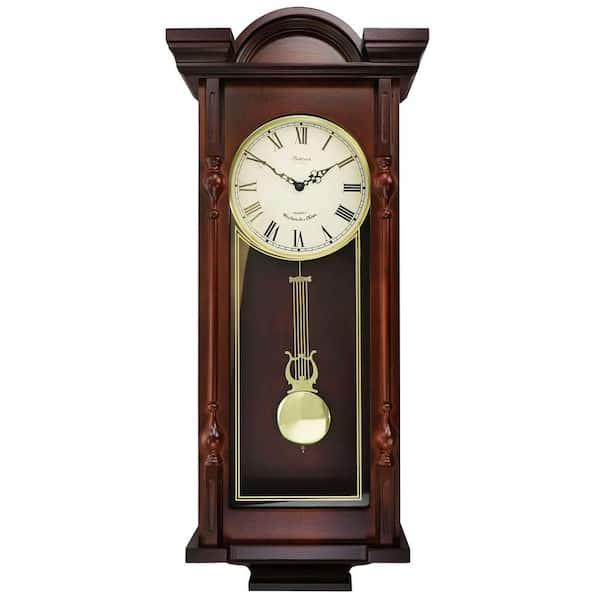This image depicts an antique-style wall-mounted grandfather clock made from dark brown, likely mahogany or cherry wood. The clock features a rectangular shape with an elegant wooden arch at the top, complemented by intricate carvings and extensions or wings on the sides. Its large white face is adorned with black Roman numerals and detailed with a gold trim around the edges. The minute and hour hands are black. Dangling below the clock face are metallic chimes that feed through a harp-shaped mechanism, which contributes to the clock chiming on the hour. The pendulum, situated behind glass, adds to the clock's ornate design with its gold or brass coloration. This beautiful piece, with its timeless charm, would make an excellent gift. The background appears white, offering no distractions from the intricate details of the clock itself.